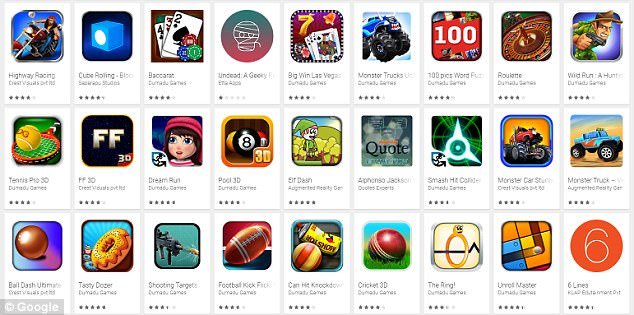The image showcases an online marketplace page where users can purchase or download a wide variety of games and apps. The selection includes word games, interactive games, football roulette, and both monster car and monster truck games. The page provides detailed information about each app, including user ratings. While most of the apps have favorable reviews with four-star ratings, one particular app stands out with a significantly lower rating of just one star, indicating a lack of popularity among users. The names of the apps are not clearly visible in the image, making it challenging for non-gamers to recognize them, although avid gamers might find them instantly familiar.